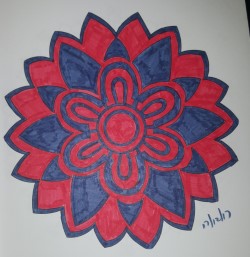This photograph features an intricate drawing of a flower set against a gray background. The flower, the main focus of the image, exhibits a complex design with alternating petals in vibrant shades of red and blue. Starting from the outer edge, the first layer of petals is blue, followed by red, and this color pattern repeats towards the center. The artwork appears to be created casually, likely intended as a fun exercise rather than a professional piece. In the bottom right-hand corner, the date "17-12-17" is penned, indicating it was drawn on December 17, 2017. This date format suggests the artist is likely non-American, as it follows the day-month-year convention. There is no other text present in the image, which, along with the date notation, suggests that the drawing is not very large and might have been done in a notebook.